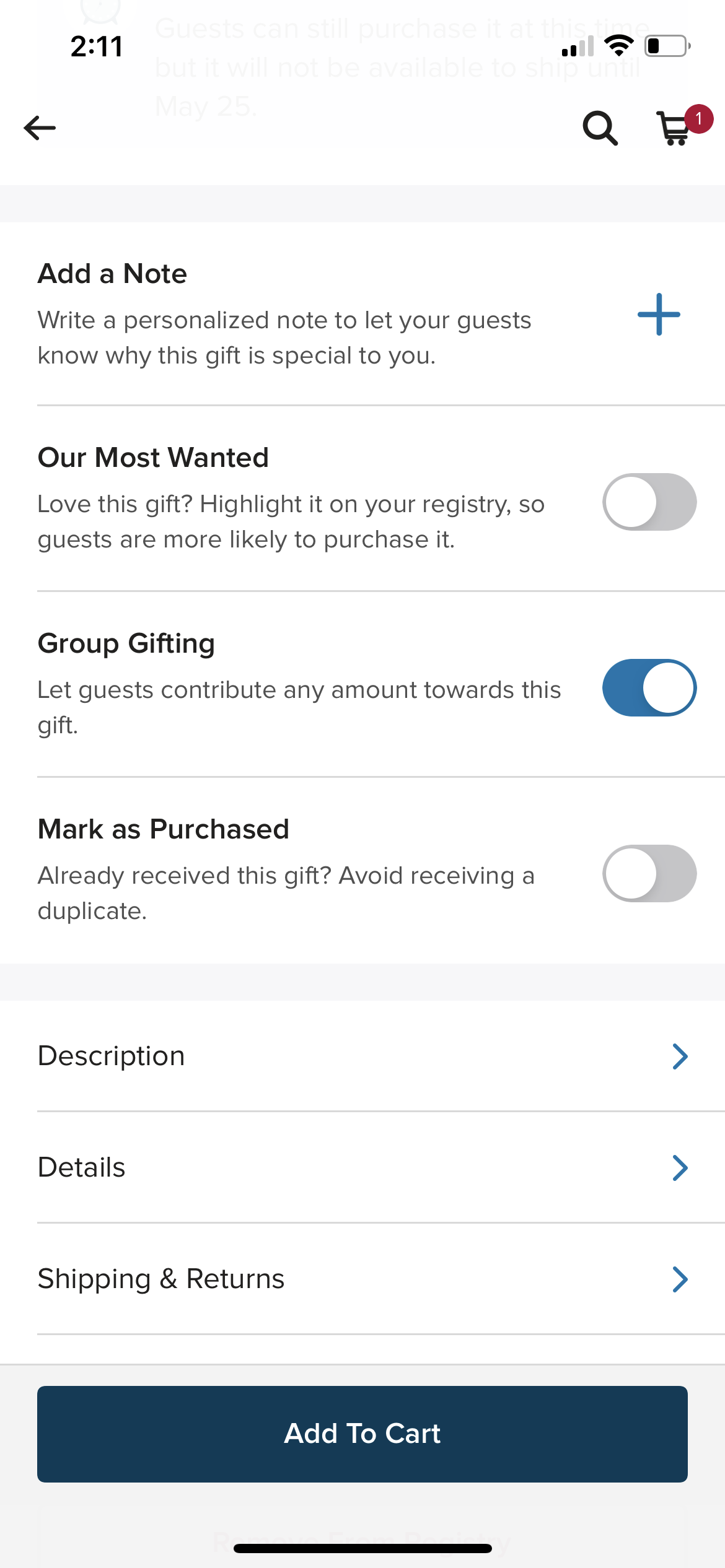This image, captured from a cell phone interface, displays a gift registry page with various interactive features. At the top, a section titled "Add a Note" invites users to "write a personalized note to let your guests know why this gift is special to you." Below that, a heading labeled "Our Most Wanted" appears, accompanied by the option "Love this gift? Highlight it on your registry so guests are more likely to purchase it," which is currently turned off, as indicated by the greyed-out toggle switch.

A prominent blue plus sign is situated above this section. The interface is neatly segmented by faint gray lines. The next section, "Group Gifting," encourages users to "let guests contribute any amount towards this gift," and this feature is turned on, illuminated in blue.

Further down, the "Mark as Purchased" section advises, "Already received this gift? Avoid receiving a duplicate," with this option turned off. At the bottom of the page, three closely grouped rectangular buttons are labeled "Description," "Details," and "Shipping and Returns," each with an arrow pointing to the right, suggesting additional information can be accessed. Lastly, a navy "Add to Cart" button provides an option to finalize the selection.